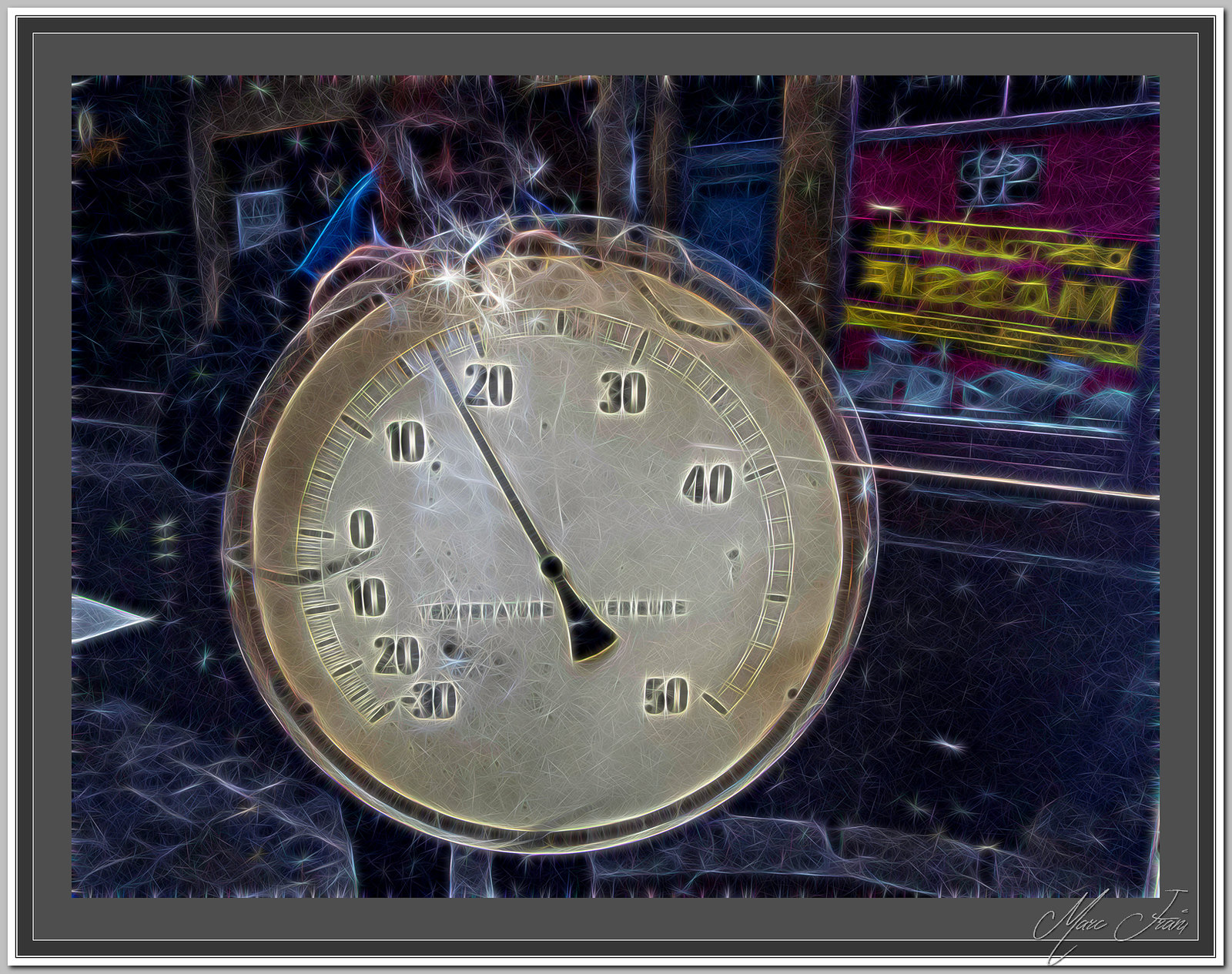This framed art piece, bordered by a sleek gray frame, features a digitally altered photograph signed by the artist in the bottom right corner. Central to the composition is a speedometer, vividly electrified with arcs of electricity radiating from its top and around its perimeter. The speedometer, marked with numerals from 10 to 50 in intervals of 10, is needle-pointed precisely at 17. 

Behind this electrifying focal point stands a man wearing an electric blue collared shirt under a black jacket, set against a bustling cityscape that resembles a shopping district. The electricity from the speedometer ascends toward his face, partially obscuring his features in a blur of static energy. In the background, a restaurant with a prominent red window and bright yellow lettering subtly melts into the scene, contributing to the overall blurred and dynamic aesthetic of the image.